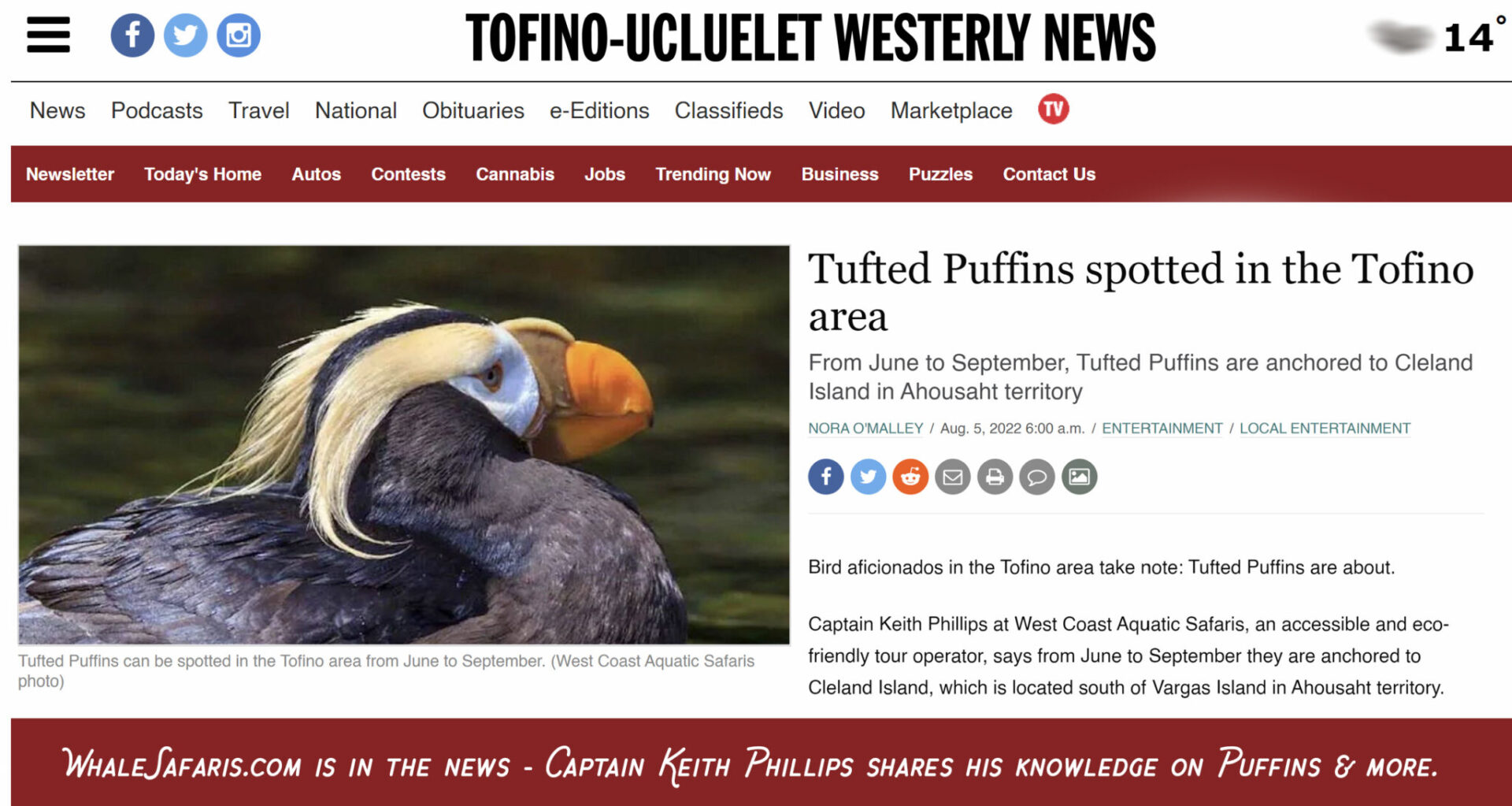**Detailed Caption:**

A screenshot displays a webpage with a clean, white background featuring various sections such as "Tofino," "Ucluelet," "Westerly News," along with a temperature indication of 14 degrees. The webpage content is organized into multiple categories including News, Podcasts, Travel, National, Obituaries, E-editions, Classifieds, Video, and Marketplace. A prominent red circle icon is labeled "TV." Additional categories on the page include Newsletter, Today's Home, Autos, Contests, Cannabis, Jobs, Trending Now, Business, Puzzles, and Contact Us.

Beside the interface details, a headline captures attention: "Tufted puffins spotted in the Tofino area." The accompanying text informs readers that from June to September, tufted puffins are commonly found anchored around Cleland Island, located in Ahousaht territory. Bird enthusiasts and aficionados in the Tofino region are encouraged to keep an eye out for these distinctive birds during this period.